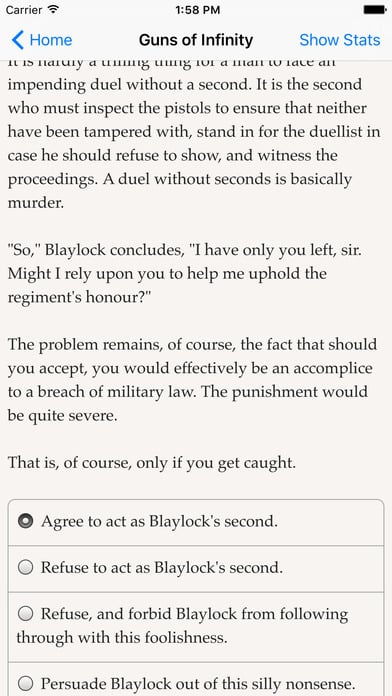A high-quality screenshot taken from a mobile device at 1:58 p.m., as indicated by the status bar at the top of the screen. The status bar shows the word "carrier" with a full battery icon and a black Wi-Fi symbol. Below the status bar, the blue navigation bar displays the "at home" option and a back arrow, with black icons representing "Guns of Infinity." The screen's background is tan with black text.

The visible portion of the text reads: "This is impending duel without a second. It is the second who must inspect the pistols to ensure that neither have been tampered with, stand in for the duelist in case he should refuse to show, and witness the proceedings. A duel without seconds is basically murder. So Blakecock concludes, 'I have only you left, sir. Might I rely upon you to help me uphold the regiment's honor? The problem remains, of course, the fact that should you accept, you would effectively be an accomplice to a breach of military law. The punishment would be quite severe. That is, of course, only if you get caught.'"

Below this narrative, there are four text box options for the user to choose from, each separated by a thin gray line. The options are as follows:
1. "Agree to act as Blakecock's second" (indicated with a black circle next to it).
2. "Refuse to act as Blakecock's second."
3. "Refuse and forbid Blakecock from following through with this foolishness."
4. "Persuade Blakecock out of this silly nonsense."

No other items or notable elements are present in the image.